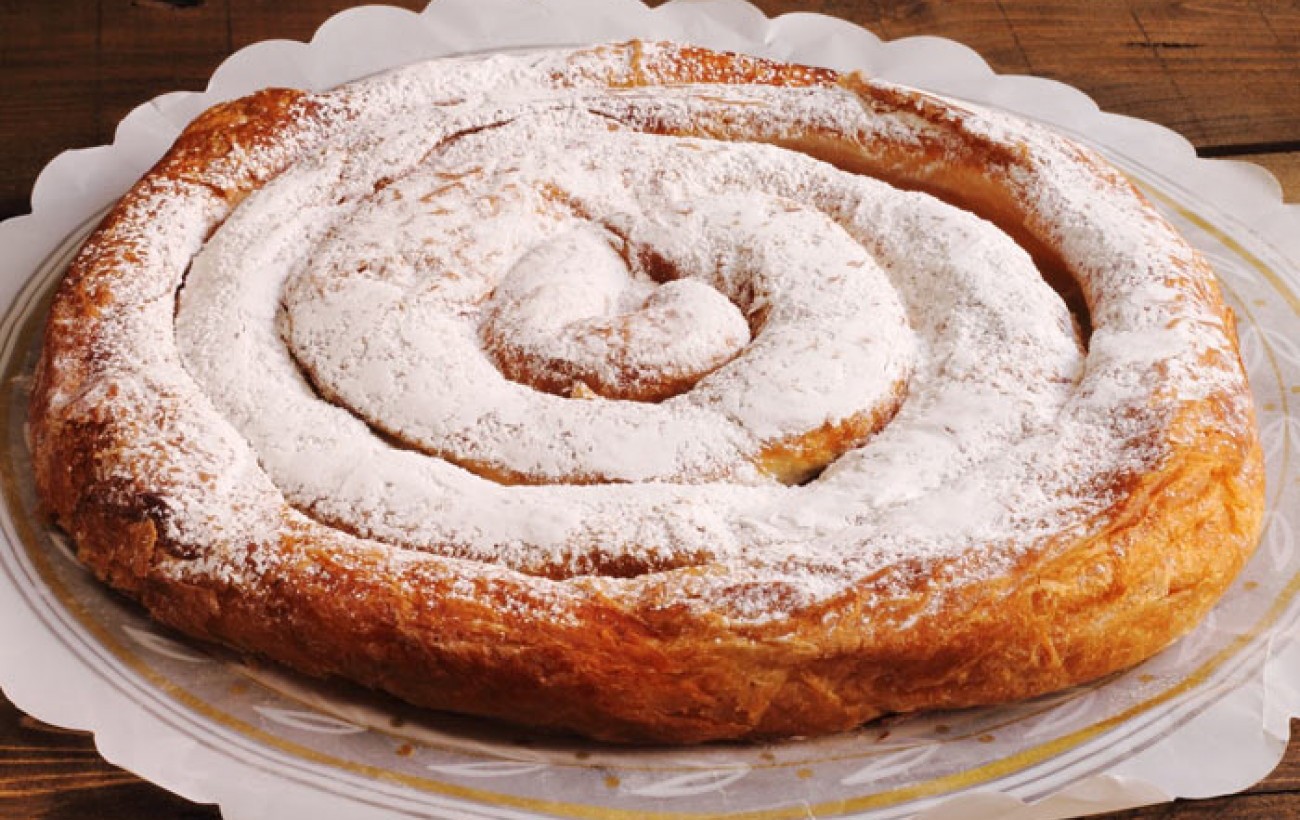This close-up photograph showcases a large spiral-shaped pastry that bears a resemblance to both a cinnamon swirl and a funnel cake. It boasts a rich, brown and golden hue, and features a flaky texture. The pastry is generously dusted with powdered sugar, with a heavier concentration towards the center, tapering off towards the edges. The pastry is presented on a clear transparent plate, which rests on a white paper mat adorned with a gold circular pattern. This setup is placed on a wooden table, the grain of which is visible at the corners of the image. There is no text or photographer credit in the image.